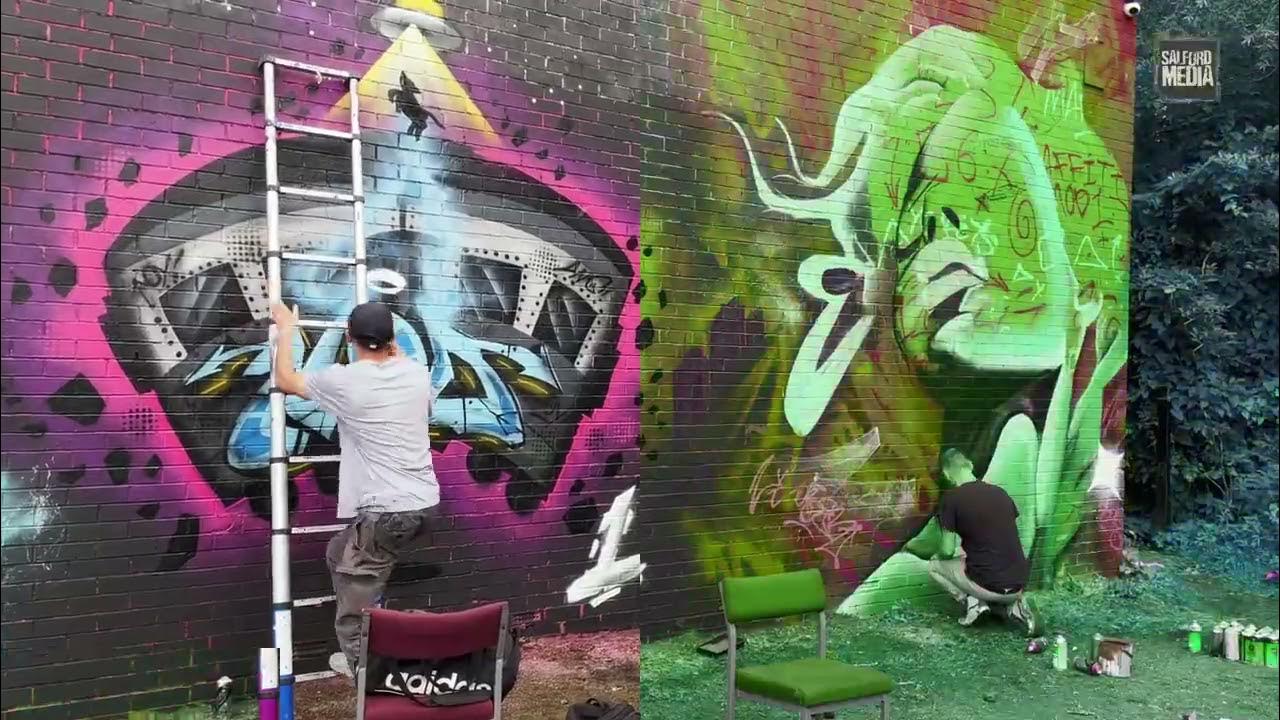The image captures an outdoor scene where two artists are working on separate colorful graffiti murals on a brick wall. A man wearing a baseball cap, a white t-shirt, and grayish pants stands on a ladder, diligently painting a vibrant and abstract piece. The left mural features a structure-like design in shades of gray and silver, highlighted with hot pink and purple hues, and is topped with the image of a howling wolf. On the right, another artist, potentially the same individual, is depicted squatting near the base of the wall, painting a striking portrait of a woman with bright green skin and wild, lime green hair adorned with various symbols. The background is filled with dynamic, colorful elements that stand out vividly against the brick canvas. In the corner, a green and purple chair and a small sign inscribed with "something media" add to the eclectic urban atmosphere.